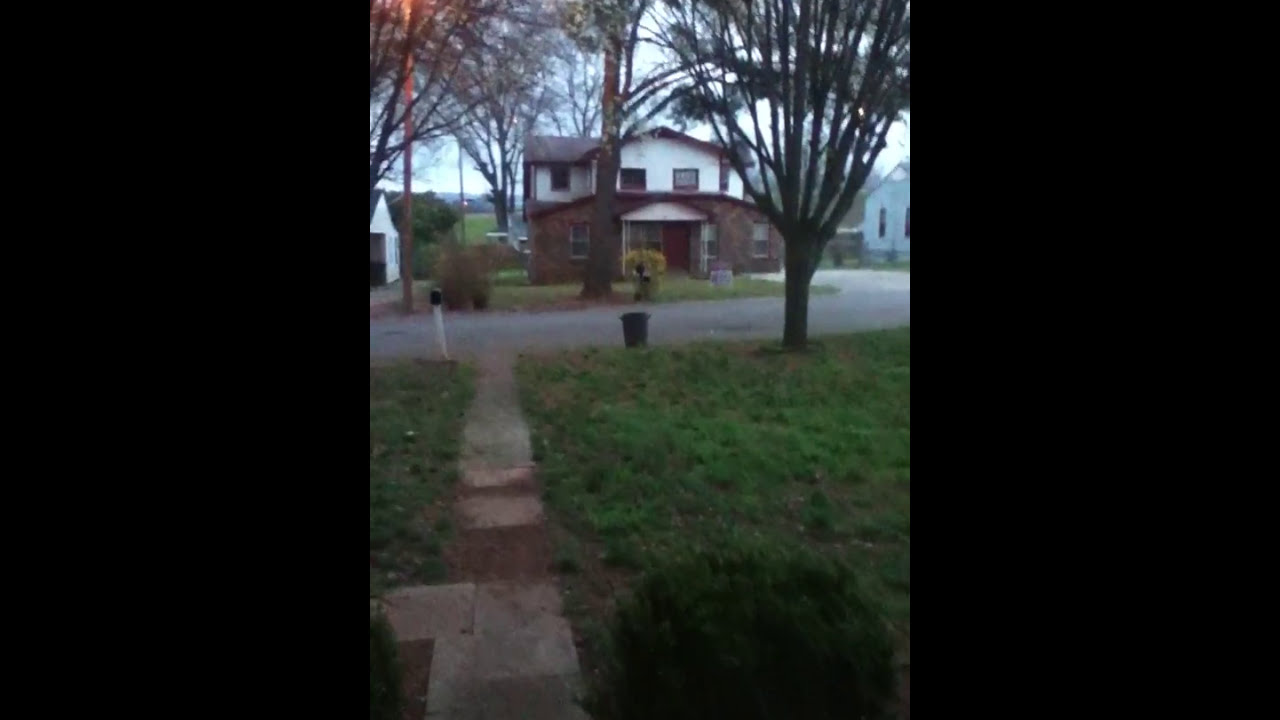The image captures a dark and overcast residential area with a light gray sky. In the center, a narrow stone brick pathway leads to a light gray asphalt road. Flanking this pathway, on the right is a green lawn with a bare tree and a small gray trash can on the curb in front of it. On the left of the pathway stands a white post supporting a black mailbox. The foreground features a grassy yard with a green bush in the lower right-hand corner. Across the street, a two-story house with a brick lower half and white-paneled upper half stands prominently, featuring a gray roof. The house has a curved driveway and is surrounded by a few mostly bare trees. The sky appears light gray, devoid of clouds or sunlight, but the thick black borders on either side of the image frame the scene distinctly.